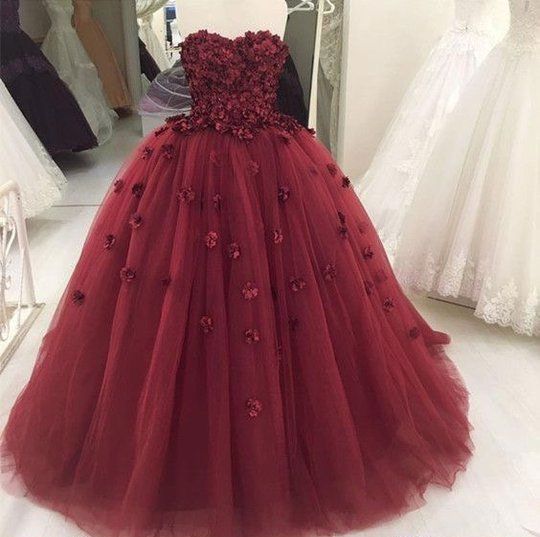In a well-appointed bridal shop, a striking burgundy strapless evening gown commands the center of the scene. The dress, made of rich taffeta, is adorned from top to bottom with intricate flower petals, giving it a ruffled and luxurious texture. The gown's voluminous skirt flows gracefully, exaggerated by its puffiness and scattered floral decorations. Beneath the gown, it's difficult to discern what it is resting on due to its fullness, but it may be draped over a mannequin. The store setting becomes evident with diverse wedding and party dresses flanking the burgundy gown. On the right, two white wedding dresses with their delicate bottoms peek into view, while on the left, a collection featuring white, beige, and a distinctive black dress add contrast. The scene is set on a white-tiled or possibly white-wood floor, adding an elegant backdrop, complemented by a white railing on the left, hinting at an upper level in the shop. In the background, more dresses hint at the variety and splendor of the bridal store's collection.